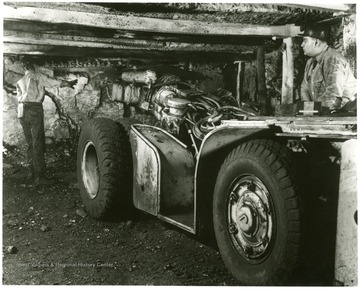In this black and white photograph, likely from an old mining operation, two men in hard hats are positioned near a low, heavy-duty vehicle with thick tires and no roof. The man on the right side of the vehicle looks back towards another man who is deeper within the cavern-like tunnel on the left. This second man has his hand resting to the side. The vehicle, possibly fitted with a drill or similar equipment, seems specially designed for work within the tunnels. The tunnel itself has wooden planks and crosswise timbers reinforcing the structure. The scene, set at the entrance of what appears to be a mine, captures the rugged, industrial essence of early mining endeavors.